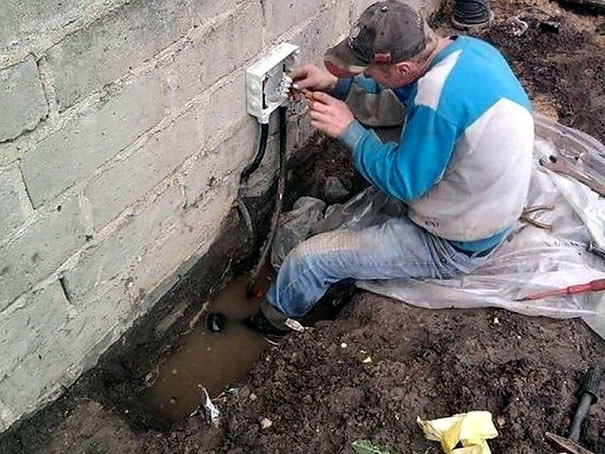A man is intensely focused as he works on an electrical circuit box connected to a pale gray brick wall. He is seated on a plastic tarp that is spread out over a muddy area, with a puddle of water partially submerging his black boots. He wears a long-sleeve blue and white shirt, blue jeans, and a gray cap. Both of his hands are occupied with something inside the white box, from which wires are protruding. Around him, a variety of tools are scattered, including a wrench, pliers, and a hammer. In the bottom right corner, there's a hint of yellow material—possibly paper or cloth—that he might need for his work. The scene conveys a sense of gritty, hands-on labor amidst less-than-ideal conditions.